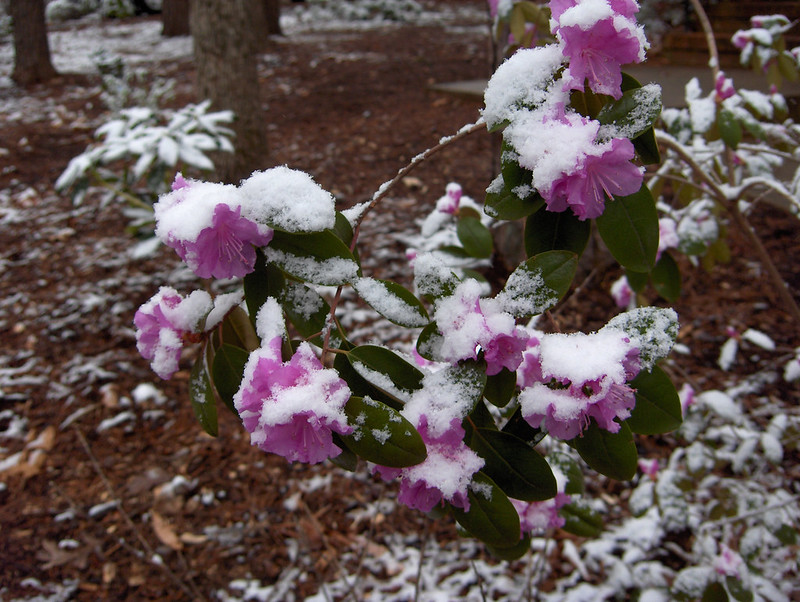The photograph is a color image taken outdoors on a dull, overcast day, using natural light. The square image primarily showcases a plant with purple flowers and rich, dark green leaves. Both the flowers and leaves, including their long filaments and thick texture, are covered in a light layer of snow, indicating a recent snowfall. The ground is primarily covered in brown wood chips, leaves, and pine needles, with some areas showing exposed bare patches, especially in the upper center and lower left corners. In the background, several tree trunks are visible, also dusted with snow. The lower right corner and upper right corner of the photograph show heavier snow accumulation. The scene captures a tranquil, wintry garden moment, devoid of people, animals, or any textual elements.